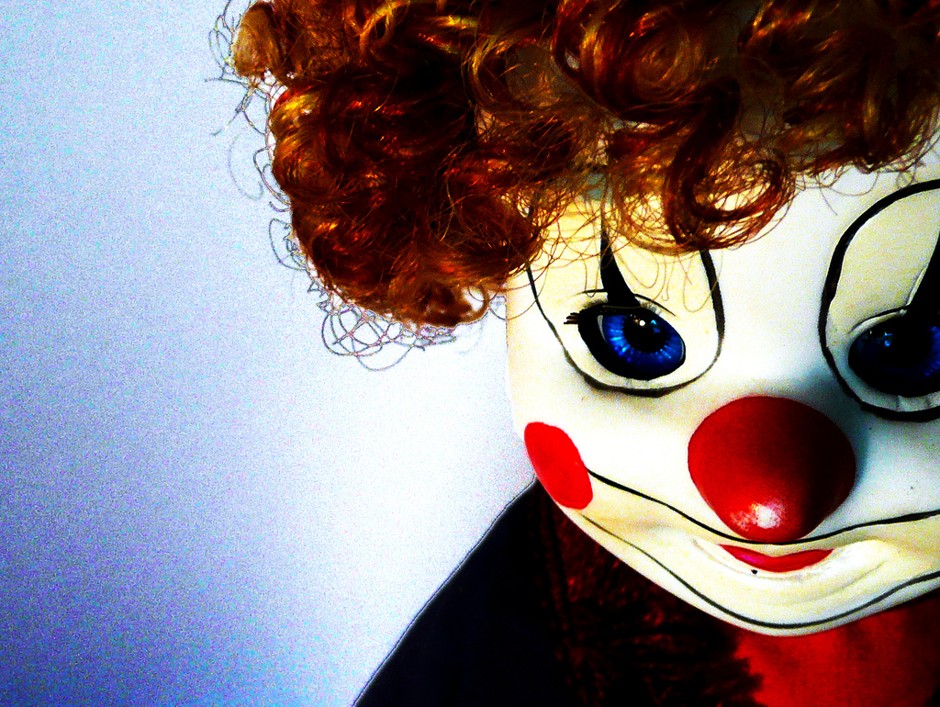The photograph is a close-up of a doll's face prominently positioned on the right side of the image. The doll has a clown-like appearance with distinctive, large, curly red hair and pale white skin. Its violet or dark blue eyes are striking, with long eyelashes that add to its eerie expression. The face is adorned with traditional clown makeup, including a red nose, circular red cheeks, and red lips outlining a smile. The background is a grainy, noisy mix of blue and white, with the light intensity stronger at the center and fading towards the edges, adding to the image's unsettling atmosphere. The figure is wearing a black and red sweatshirt, contributing to the doll's overall creepy aesthetic reminiscent of a character like the Joker. The low resolution and noisy quality of the photograph enhance the unsettling, creepy vibe of the doll's visage.